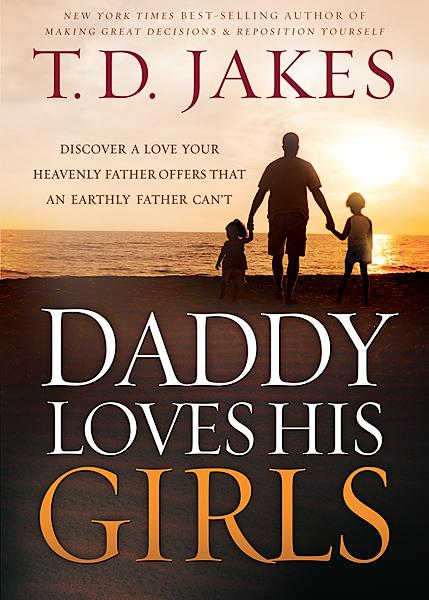The book cover showcases a serene beach scene at sunset, with a New York Times bestselling author heading the title. T.D. Jakes, known for "Making Great Decisions" and "Reposition Yourself," is prominently displayed in red at the top. Beneath his name, the cover reads, "Discover a love your heavenly father offers that an earthly father can't." 

The central image features a father figure walking on the sand, holding the hands of two children—the smaller child is on his left, and the slightly larger child on his right. They are facing the ocean, its water reflecting the bright orange hues of the setting sun. The day's last light creates a tranquil atmosphere as it glows on the water. The children, both wearing shorts, stride alongside their father towards the horizon under a partly cloudy sky.

At the bottom in bold uppercase letters, the title "Daddy Loves His Girls" is divided into "Daddy Loves His" in white and "Girls" in orange. This touching depiction emphasizes the profound bond between the father and his daughters as they embrace this peaceful moment together.